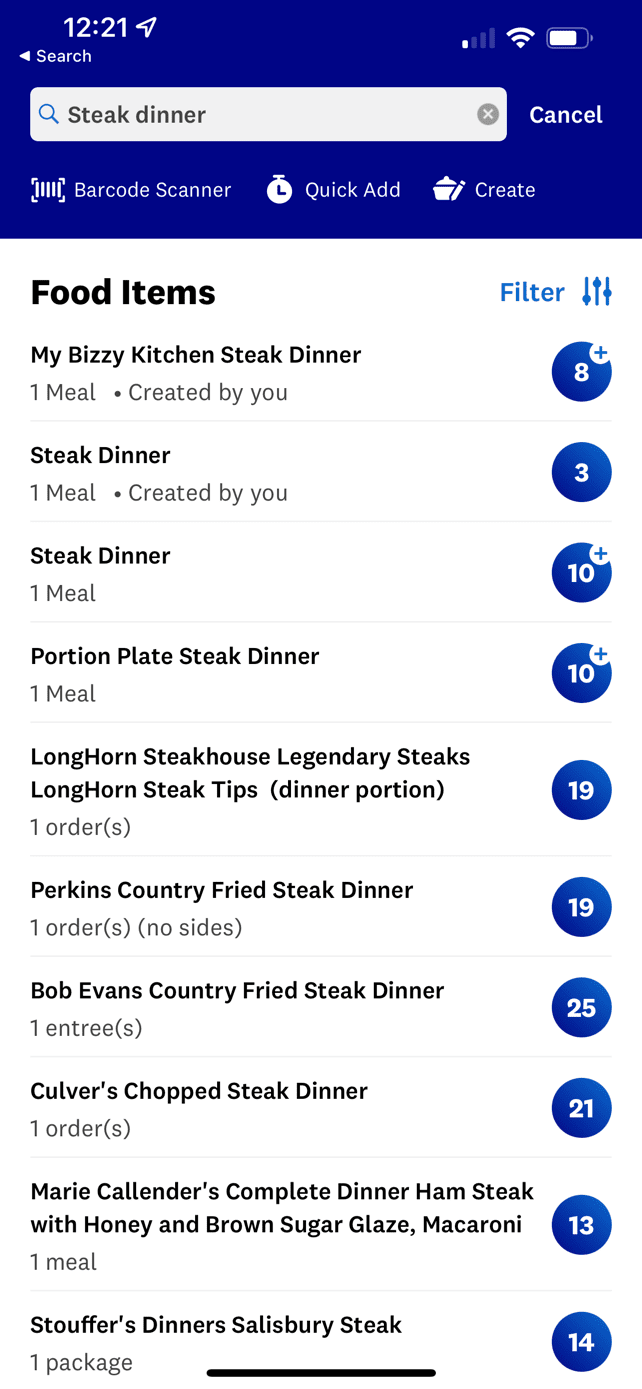On a smartphone screen, the top section displays a blue background with a white left sidebar. The time reads "12:21" with a right-pointing arrow next to it. Below, a left-pointing triangle is labeled "Search." The signal indicator shows a single white bar, indicating low service, but the Wi-Fi icon shows all bars, indicating a strong connection. The battery icon, displayed in white, is over 75% charged.

Beneath these indicators is a white rectangular search box. On the left side of the box, there is a blue magnifying glass icon, and next to it, the words "steak dinner" in black text with a gray circle containing a white "X" beside it. On the right side of the box, the word "Cancel" is written in white.

Following this, a white text reads "Barcode Scanner, Quick Add, Create" against a black background. The screen is divided into two sections.

On the left side, the heading "Food Items" is in black text. Listed under this heading are several entries about "steak dinner," each followed by varying descriptions and portions:

- My Busy Kitchen, Steak Dinner, One Meal Created by You
- Steak Dinner, One Meal Created by You
- Steak Dinner, One Meal, Portion, Place
- LongHorn Steak, Legendary Steaks, LongHorn Steak, Tips (Dinner Portion), One Order
- Perkins Country Fried Steak, Dinner, One Order, No Sides
- Bob Evans Country Fried Steak, Dinner, One Entrée
- Culver's Chopped Steak, Dinner, One Order
- Marie Callender's Complete Dinner, Ham, Steak with Honey and Brown Sugar Glaze, Macaroni, One Meal
- Sofra's Dinner Style, Mary's Steak, One Package

A horizontal black line separates this list from the right side of the screen, where a blue "Filter" button is located. Various blue circles display white numbers, representing different quantities:

- 8
- 3
- 10
- 10
- 19
- 19
- 25
- 21
- 13
- 14